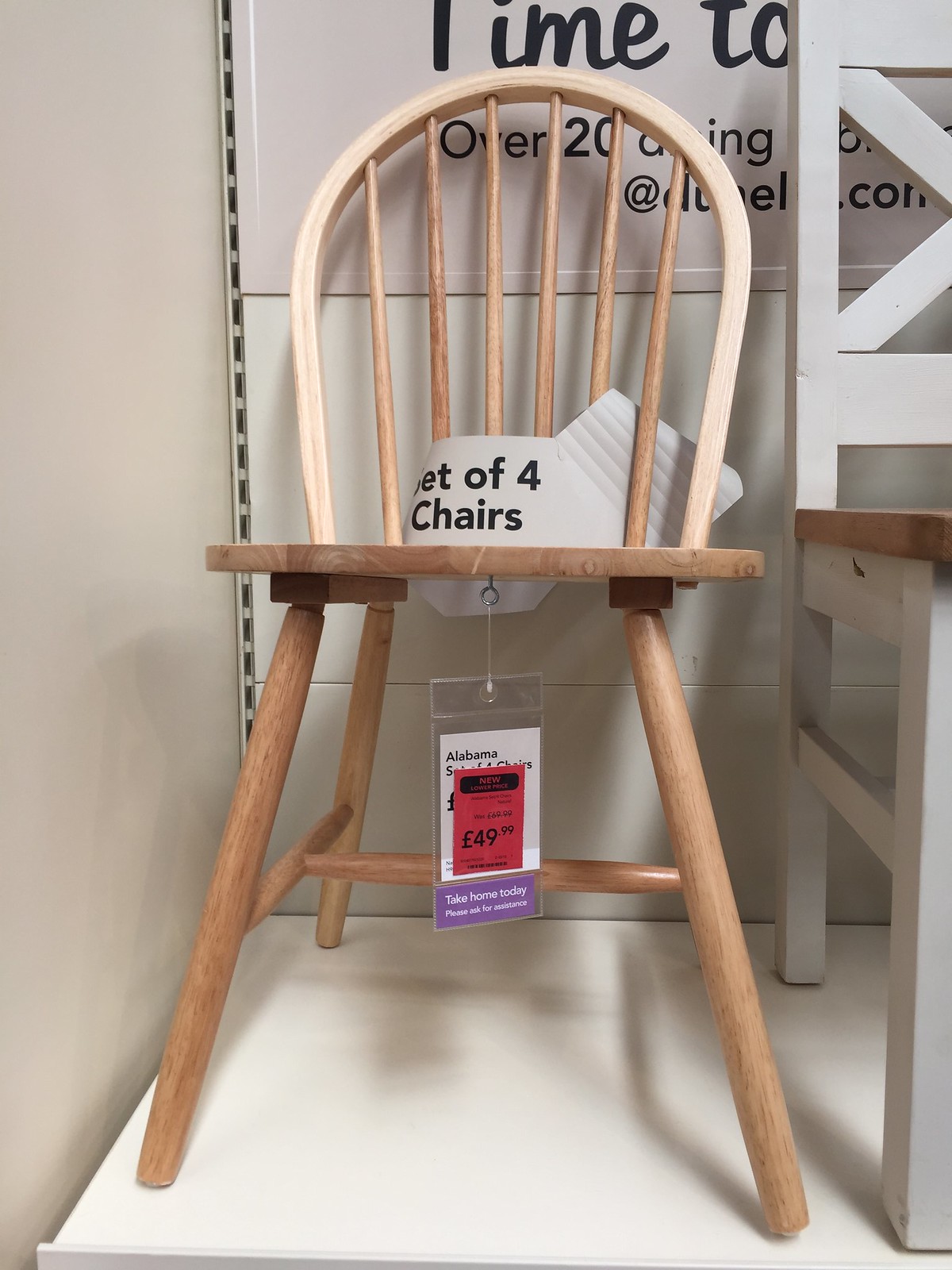The image depicts a prominently displayed wooden chair in a store, occupying most of the frame. The chair features a natural light tan wooden color with round and smooth characteristics. Its backrest consists of a thick oval-shaped wooden piece supported by six vertical, evenly spaced poles. There is a noticeable white paper sign attached to the backrest, albeit bent, indicating that it is a "set of four chairs," although part of the text is obscured. The chair’s four legs are reinforced by H-shaped wooden connectors.

Hanging from the underside of the chair is a red tag with the price marked as €49.99. Additionally, a larger white tag with the text "Alabama" is partly visible, with the rest blocked by a small red paper. Below these tags, a purple tag reads "Take home today, please ask for assistance." The chair is displayed on a plain white shelf or platform typical of store showcases.

To the right of the wooden chair sits another chair of a different style and white color, which is more angular in design. In the background, partially visible signage includes the phrases "time to" and "over 20 something something.com".